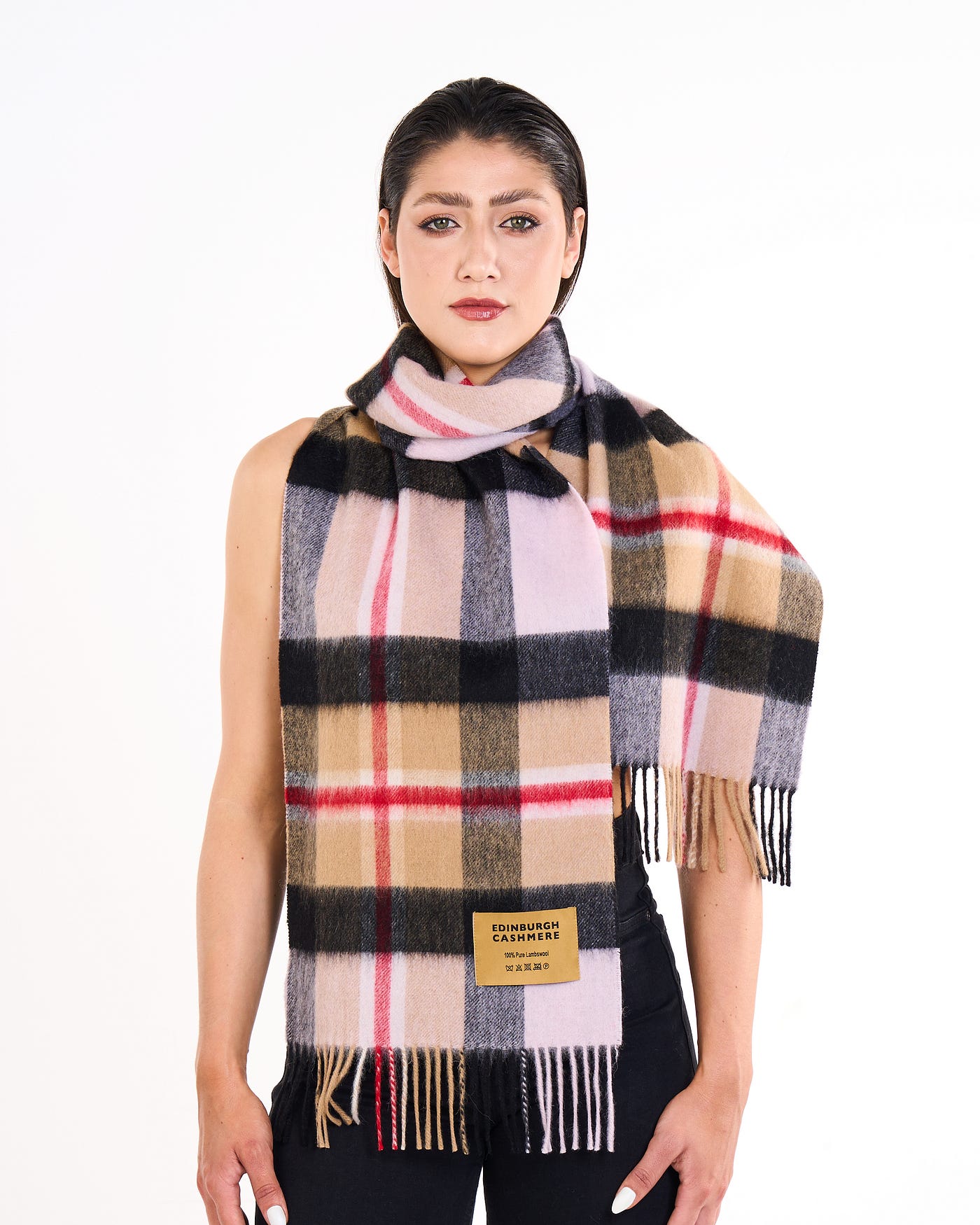The photograph is a sleek and minimalistic fashion advertisement featuring a slender woman of possibly Asian or Eurasian descent, standing against a plain white background. She is showcasing a large scarf with a classic Burberry-like pattern in tan, black, white or cream, and red. The scarf, labeled with a tag that reads "Edinburgh Cashmere," is prominently displayed, crisscrossed around her neck and draping down to cover her torso and the upper half of her left arm. Her right arm hangs straight down at her side, exposed. She is wearing black pants, her attire monochromatic except for her bold, dark red lipstick. Her black hair is slicked back, drawing attention to her meticulously polished white nails and an air of sophistication enhanced by full makeup, brown eyes, and a poised, fashion-forward demeanor.